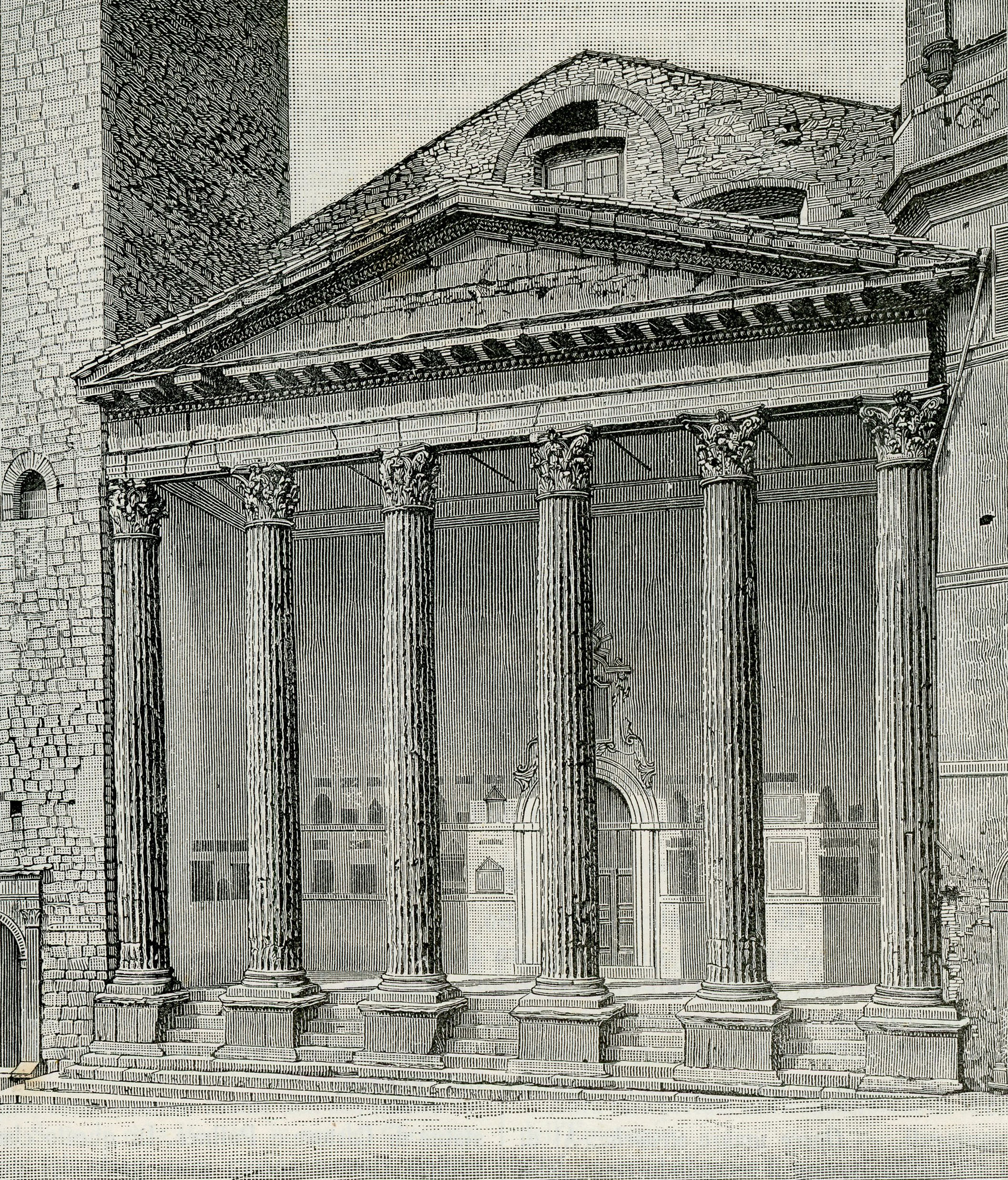The image depicts a highly detailed hand-drawn or possibly charcoal sketch of a grand Roman-style building. This black and white illustration showcases a monumental structure with six towering, intricately designed stone and brick pillars at the forefront. Each pillar, likely about 20 feet tall, rests on square bases and supports a triangular pediment roof, with another triangular section above containing a stone surface composed of small, arranged pieces. This area also features a circular stone design framing a square window.

The building has a centrally located staircase leading up to a large archway that serves as the main entrance, potentially adorned with a wooden door. To the left side of the image, another wide and tall column extends beyond the frame's top, albeit without a visible peak, and includes a couple of arch-shaped windows. The entire scene is set against a gray sky, emphasizing the architectural details of the structure. This grand facade is punctuated with various windows and a tower-like structure on the upper parts, enhancing the complex and ancient aura of the building, a testament to exquisite craftsmanship in stone and brick.